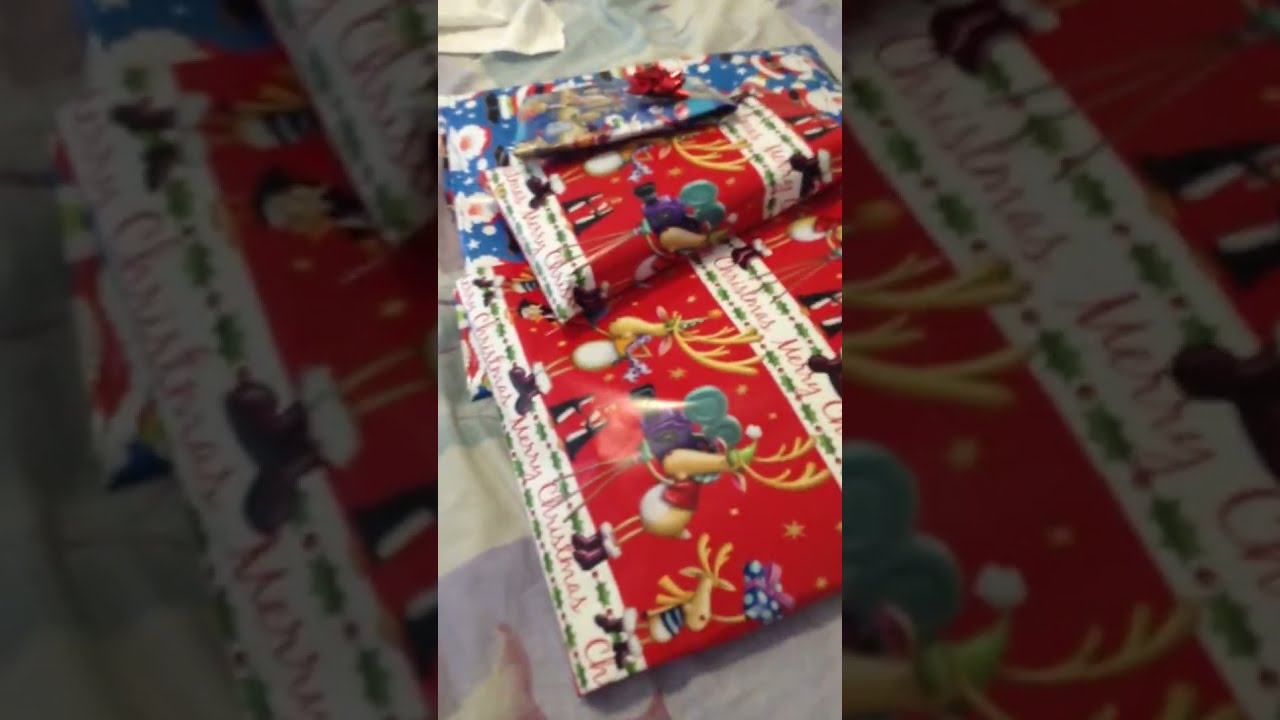The photograph captures a hospital room with a man centrally positioned, wearing a white, short-sleeved V-neck t-shirt adorned with a black and white design, and khaki shorts. He appears worried or serious, looking down at his phone or an object, seated cross-legged on a bed. The room features predominantly yellow walls, a blue mattress, and a window with blinds in the background. In addition, there is an IV post with cords attached to the bed, as well as various bags and personal belongings scattered around. Behind the man, only the legs of two other individuals are visible, seated on an adjustable hospital bed near a window, with a reflective closet door capturing the man's reflection on one side. The overall scene is devoid of any text or inscriptions.